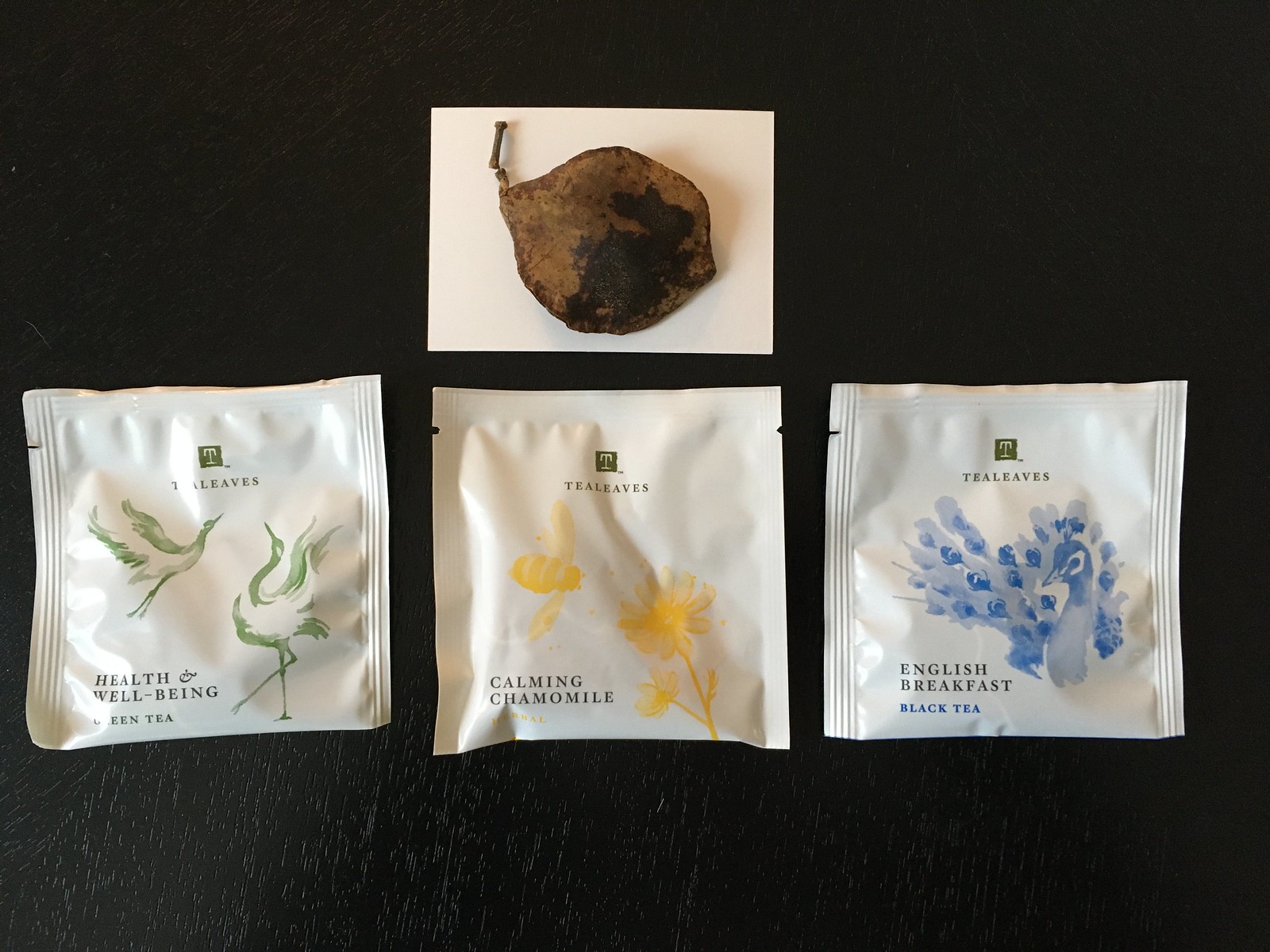This overhead image captures a meticulously arranged display of three white, square tea packets set against a black wooden surface that lightens slightly at the bottom and features tiny, black notches. Each packet bears the same green logo—a green box with a white letter 'T'—and the label "tea leaves" at the top. The variations among them lie in their designs and flavors: 

1. The packet on the left reads "health and well-being, green tea" and is decorated with two green watercolor herons, one flying and the other standing.
2. The middle packet is labeled "calming chamomile" and features a yellow bee approaching a yellow flower.
3. The packet on the right displays "English breakfast, black tea" with a blue illustration of a male peacock, its tail fanned out stylishly.

At the top center of the image, positioned on a white piece of paper, is a used teabag. The teabag, exhibiting a darker, wet lower half filled with dark tea particles and a lighter, dry top half, has a stem hanging from its left side. The detailed nuances of the scene provide a harmonious yet varied portrayal of different tea selections.